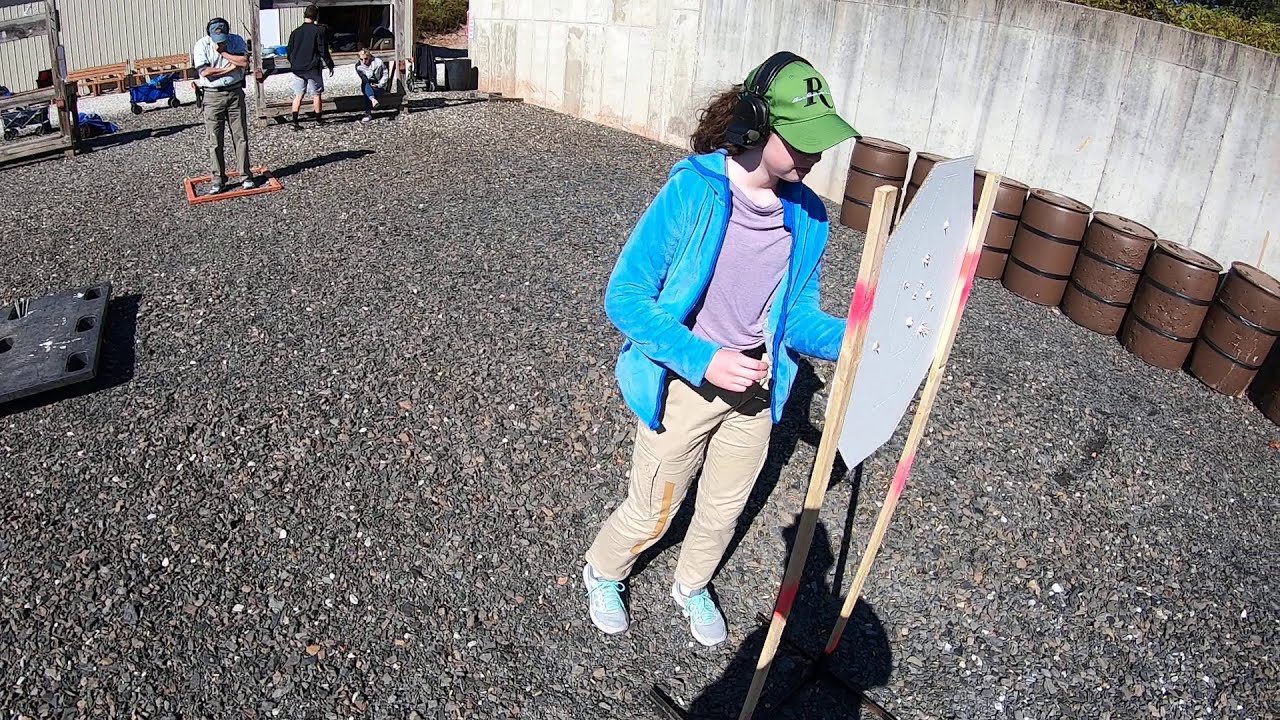In the image, a detailed scene at a shooting range unfolds. Central to the picture is a young girl with light skin, donned in a light blue hoodie over a purple t-shirt, beige or brown cargo pants, and white and blue sneakers. She stands on a gravel ground in front of a hexagonal paper target mounted on two wooden sticks. The girl, sporting a green cap with the letter 'R' and curly, shoulder-length brown hair, wears large black safety headphones. To her side are large brown barrels adorned with blue and black stripes. Behind her, a man under a rectangular or square structure is observing the ground, wearing a cap and similar headphones. In the backdrop, additional individuals, including one seated and another walking, are within a gated area featuring concrete walls and shooting stands.